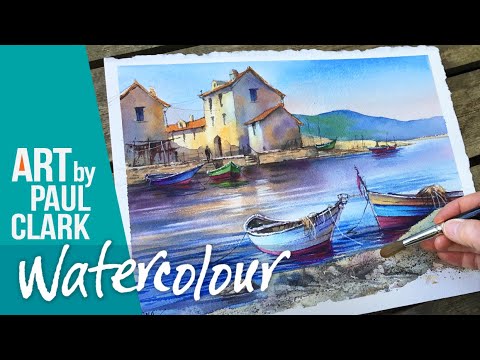In this photograph, we see an artist meticulously creating a watercolor painting on a wooden or picnic table. The upper left corner of the image features the text “Art by Paul Clark” in white against a bluish background, and at the bottom, it reads “Watercolor.” Dominating the right-hand side, the artist’s hand holding a brush is working on a picturesque scene that appears inspired by a coastal Italian village. 

The painting shows a serene body of water with a reflection of orange from the sun, encircled by small fishing boats. Two boats in the foreground, one yellow, blue, and red and another white and red, rest near the shore where the artist's hand is placed. Further into the distance, a red and white boat can be seen alongside a green and red boat and a blue and red boat.

The backdrop of the scene includes a white stucco-style two-story house, characterized by its red roof and small, old-fashioned windows, suggesting it is an aging structure. A person can be seen walking down steps towards the water, adding a human element to the tranquil setting. Off in the distance, majestic mountains rise, completing the picturesque landscape that the artist is capturing.